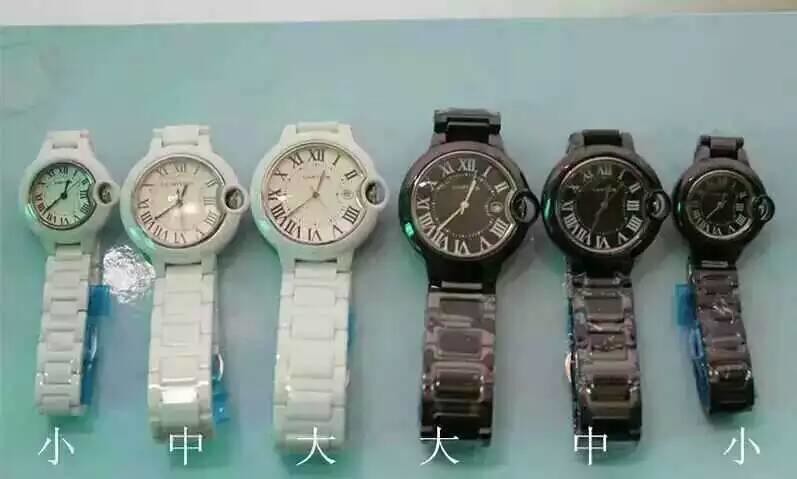This image showcases six elegant wristwatches, meticulously arranged in a row. The watches exhibit slight variations in size but are strikingly similar in design. 

Starting with the watch on the far left, it features a sleek white metal case with a matching white bezel encircling the face. The dial is adorned with classic Roman numeral markers from 1 through 12. The white watch face contrasts strikingly with the silver hour and minute hands, along with a faint, almost subtle, second hand. A small crown on the right side of the watch is visible, presumably for setting the time.

To the immediate left of this watch, there is a slightly smaller version sharing the same design features. Further left is an even smaller iteration, maintaining the consistent design characteristics.

On the right side of the largest white watch is a black counterpart. This timepiece mirrors the white version in structure, boasting a black metal case and black bezel. The face of the watch is also black, with white Roman numeral markers providing a sharp contrast. The hour, minute, and second hands are all in white, ensuring legibility against the dark backdrop.

Continuing to the right, the next watch is a smaller version of the black design, followed by an even smaller one to its right. 

Beneath each watch, there is an inscription of an oriental symbol, the meaning of which remains unknown. This setup highlights not only the aesthetic harmony between the different sizes but also the intricate details and timeless design of each watch.